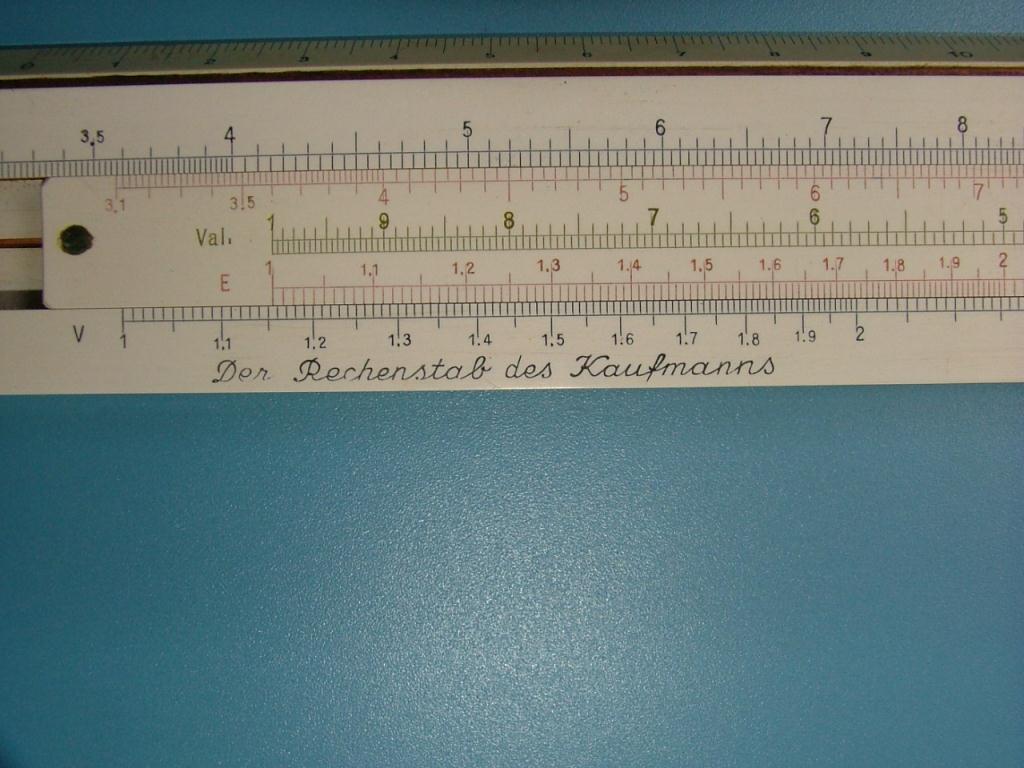The close-up image features a collection of rulers arranged horizontally on a slightly glossy yet matte textured surface painted in a metallic gray-blue color. The texture of the background is visibly distinct, adding depth to the photograph. The rulers, whose material might be either wood or metal, display various measurement standards. Some rulers are marked with inch increments, such as 4, 5, 6, 7, and 8, while others show metric calibrations, including precise measurements like 1.0, 1.1, 1.2, and 1.3 centimeters. The diversity in the calibration and design of the rulers offers a detailed and intriguing visual study of different measuring tools.